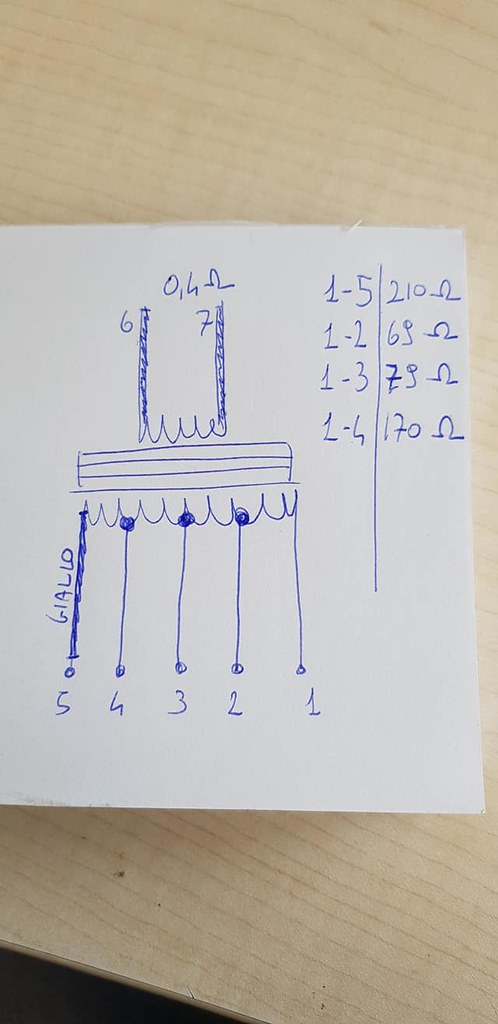This photograph showcases a white piece of paper lying on a tabletop with a light wood grain, resembling birch wood. The hand-drawn diagram on the paper, created with blue ink, illustrates a transformer with multiple taps. On the primary side, pins 6 and 7 are marked, with a note indicating "0.40." On the secondary side, there are five taps labeled 1 through 5. The leftmost tap is marked with the word "GIALLO." Adjacent to the diagram, a handwritten table details the resistance measurements: 

- 1 to 5: 210 ohms
- 1 to 2: 63 ohms
- 1 to 3: 73 ohms
- 1 to 4: 170 ohms

The entire diagram and accompanying table are crudely drawn with a blue ballpoint pen, contributing to a rough and informal appearance.